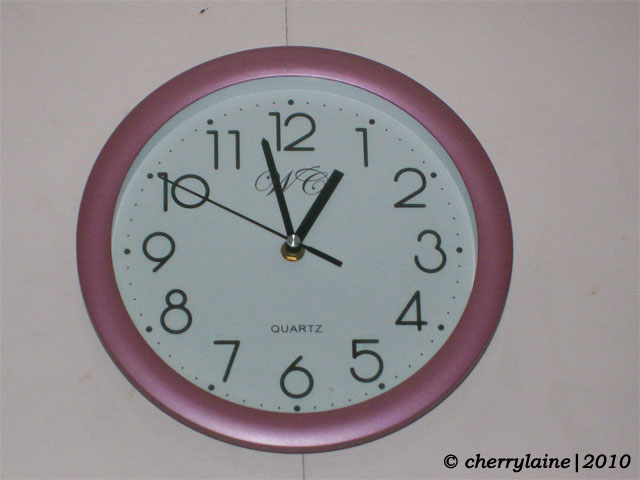The image depicts a round, pink clock mounted on a white wall. The clock's border, measuring approximately an inch in thickness, is a metallic pink, contrasting with the white face of the clock. The clock features black numbers in a whimsical, rounded font, with distinctive characteristics such as a bubbly numeral three and an exaggerated circular component in the number nine with a small tail. Both the hour and minute hands are also black.

At the top of the clock, below the 12, there is a logo in script featuring the letters "W" and "C" in an elegant font. The word "Quartz" is inscribed above the six. In the bottom right corner of the image, there is a copyright symbol followed by "Cherry Laine," separated by a vertical line, and the year "2010," all printed in black.